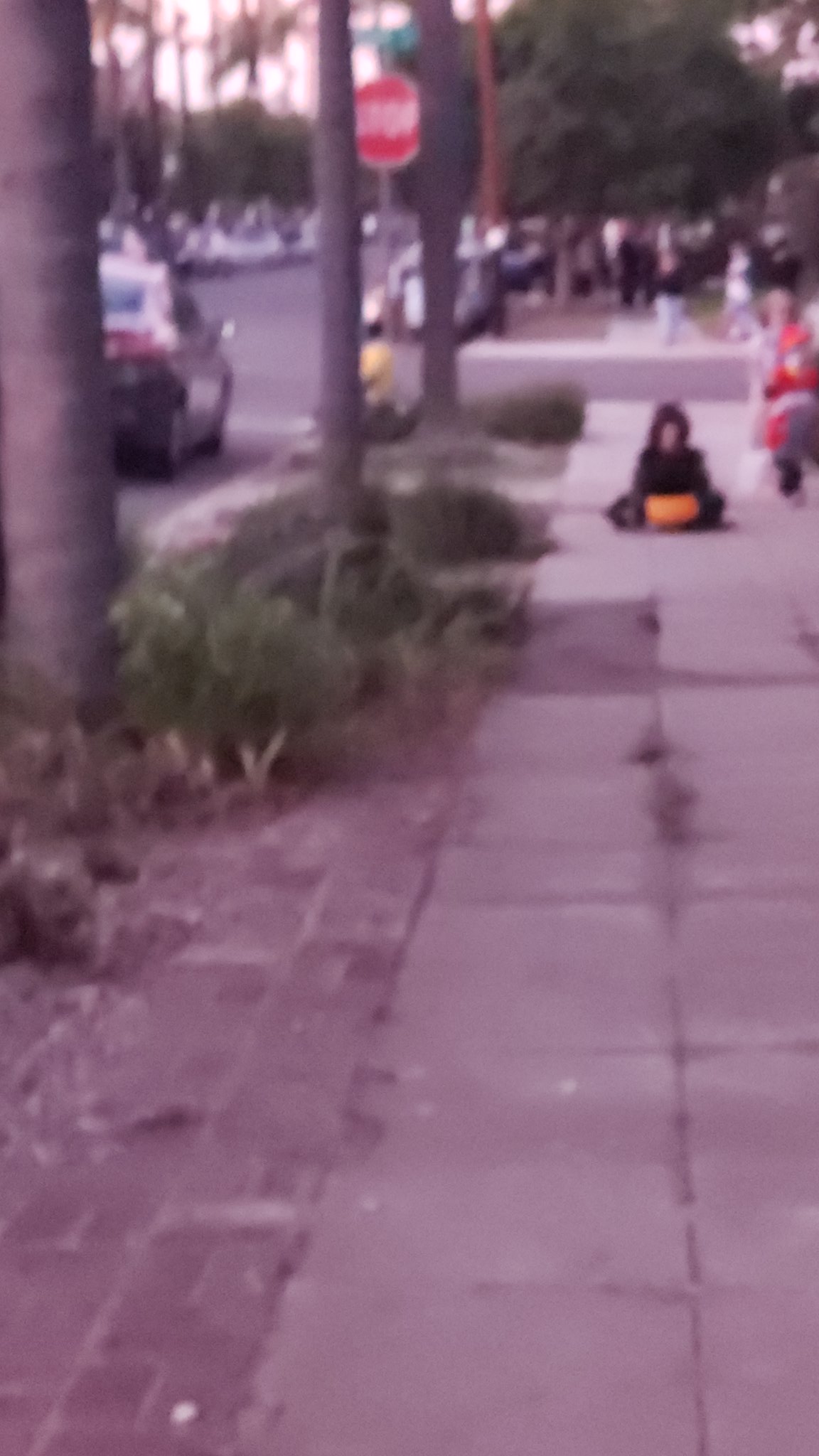This vertically arranged rectangular photo, potentially quite old and very blurry, shows an outdoor scene suffused with a lilac hue. The left side of the image depicts a street lined with palm trees leading to a red stop sign where a black car is halted. Behind this street, the broken concrete slabs of a sidewalk stretch out, bordered by brick and interspersed with several green bushes and tree trunks. Further in the distance, the sidewalk continues past another street running horizontally.

In the foreground, a child dressed in a dark black hoodie sits on an orange object that could be mistaken for the front of a sled. Nearby, a person clad in red stands close to the camera. The background reveals additional cars lining the street and a grassy area to the right, scattered with more palm trees. A few people are visible walking along the sidewalk in the distance, indirectly emphasizing the blurry and nostalgic quality of the image.